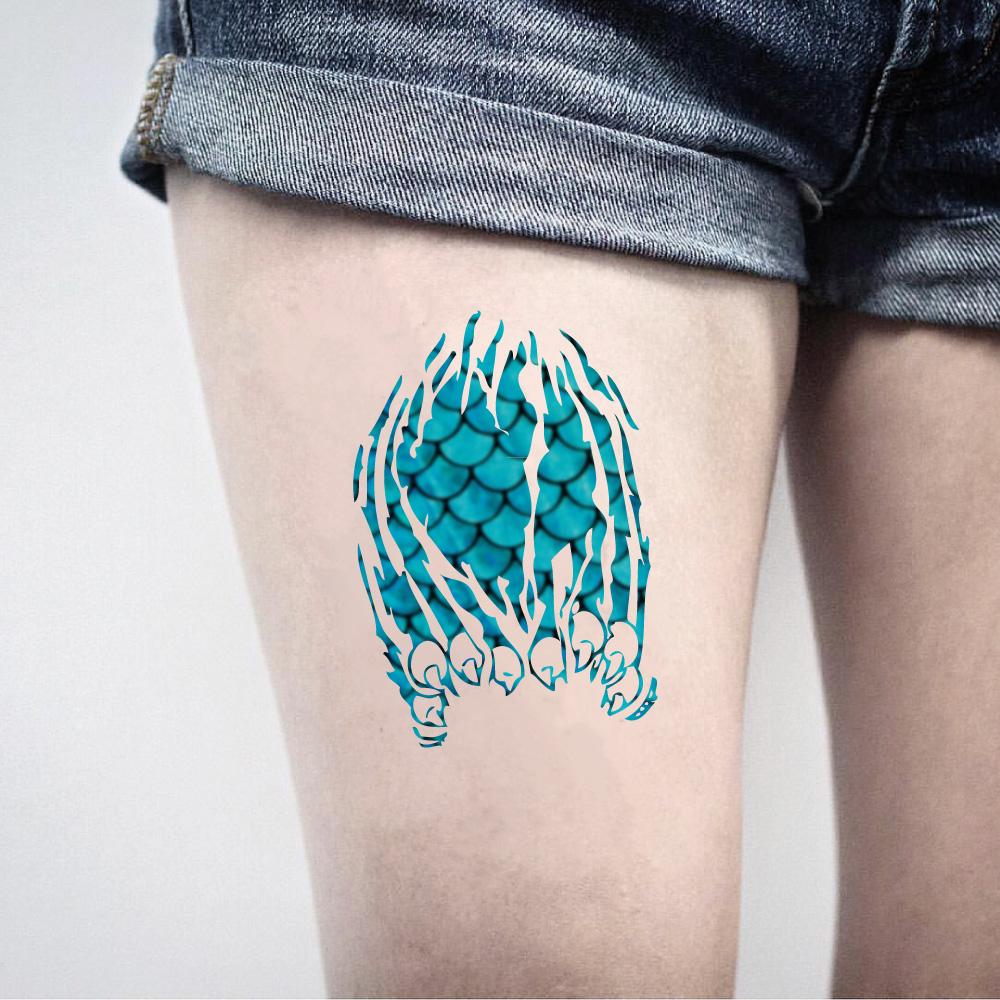The image captures a close-up of a person's thigh, predominantly the right leg, though part of the left thigh is also visible. The person appears to be wearing very short, gray jean shorts, revealing a detailed and vibrant tattoo on their pale skin. The tattoo artistically resembles scales, likely of a fish or snake, depicted in a striking teal blue color. These finely detailed scales cover most of the tattoo, transitioning into a series of sharp, white claws towards the bottom. These claws, about eight or nine in number, stretch down from the scales and seem to reach toward the knee. The realistic and intricate design of the tattoo creates an almost 3D effect, making it appear as though the scales and claws are emerging from the skin itself.